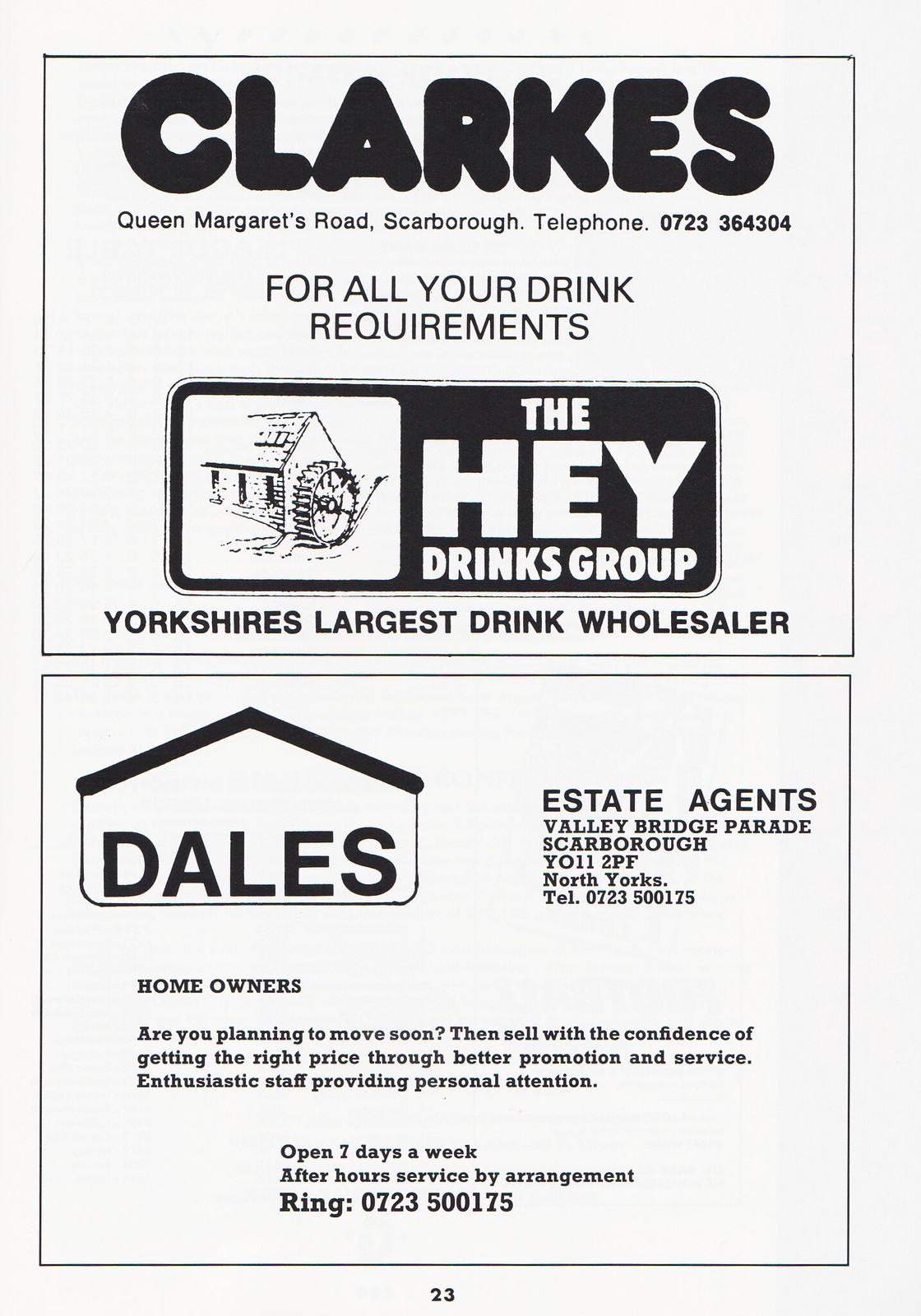The image appears to be from a page of a magazine or a newspaper, specifically page 23, as indicated by the small, black sans-serif text located at the bottom center of the page. The page contains two equally-sized advertisements, each enclosed within a thin, black border.

The upper half of the page features an advertisement for Clarke's. At the very top, it showcases the name "CLARKE'S" in large, black, bold, puffed-up sans-serif letters, with the address "Queen Margaret's Road, Scarborough," followed by the phone number "0723 364 304" in smaller text below it. Underneath, in all capital letters, "FOR YOUR DRINK REQUIREMENTS" appears in black. Next, there is an image of a water mill, a black sketch, positioned to the left, with "The Hay Drinks Group" written in large white letters inside a black rectangle to its right. At the bottom of the ad, smaller black text reads "Yorkshire's Largest Drink Wholesaler."

The lower half of the page is dedicated to an advertisement for Dales Estate Agents. The ad starts with a logo of a house outlined in black, with the word "DALES" inside it in black print. Adjacent to this logo, the text "Estate Agent, Valley Bridge Parade, Scarborough" appears, along with the postal code "Y011 2PF" and "North Yorkshire." Below this, the phone number is provided as "TEL. 0723 500175". There is a paragraph of text labeled "Homeowners," asking, "Are you planning to move soon?" and encouraging potential clients to "sell with the confidence" of obtaining "the right price for better promotion and service." The paragraph further details that enthusiastic staff provide professional and personal attention, and mentions availability "seven days a week" with "after hour service by arrangement" and instructs to "ring; 0723 500175."

Both advertisements use a combination of sans-serif and serif fonts and are surrounded by clean, thin black borders.